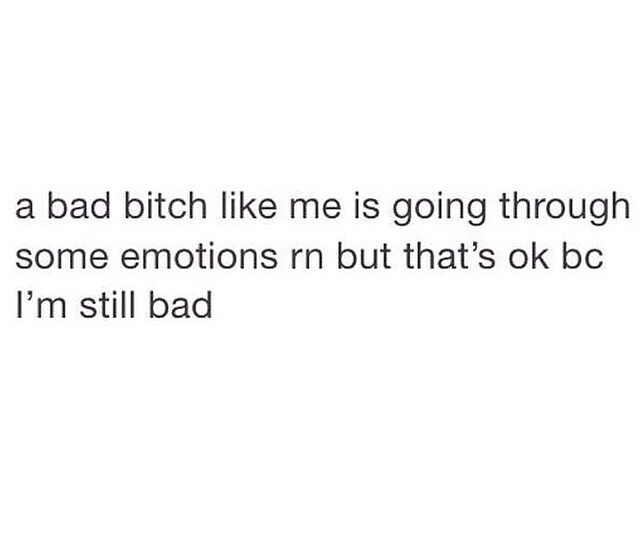This image features a stark white backdrop with a centrally positioned piece of text in bold, black letters. The text takes up a significant portion of the middle of the image and reads: "a bad bitch like me is going through some emotions, RN, but that's okay, BC, I'm still bad." Notably, the text is all lowercase, except for the capitalized "I" in "I'm," giving it a casual, conversational feel, as if it’s a personal statement or a quote. Common internet shorthand is used, with "RN" standing for "right now" and "BC" standing for "because." The entire quote is left-aligned and free of any punctuation or additional design elements, suggesting a purposefully minimalist and raw expression of emotion, possibly intended for social media sharing.